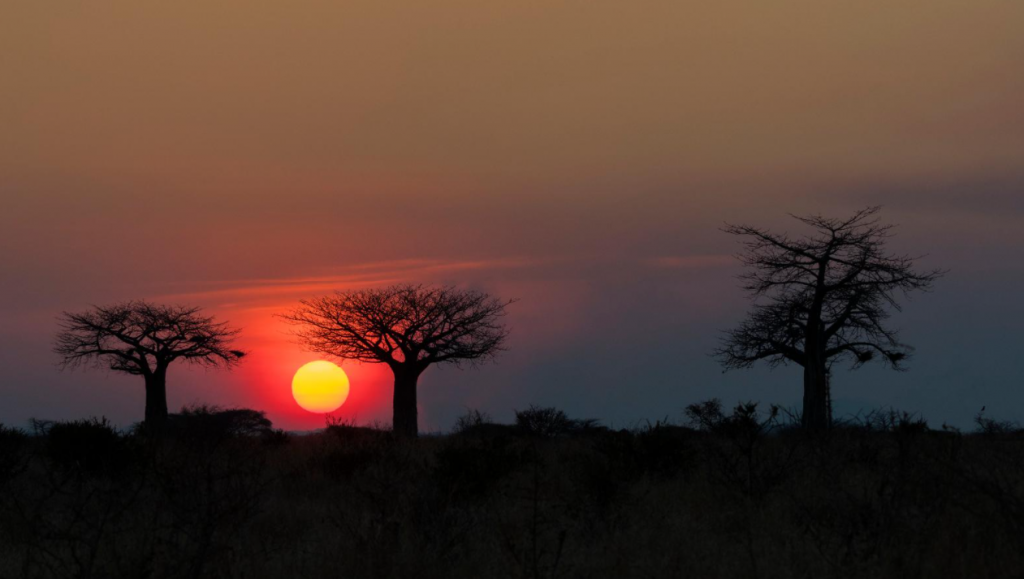The image captures a stunning sunset at nightfall, showcasing a gradient sky transitioning from light hues to purplish-pink and gray, tinged with blues, yellows, and reds. Dominating the scene, the sun appears as a large, round yellow orb encircled by vivid orange, situated slightly off-center to the left. Silhouetted against this vibrant sky are three starkly black trees, devoid of leaves, standing prominently—one to the left and two to the right of the sun. The foreground is enveloped in deep black tones, suggesting a grassy hillside shrouded in darkness. The contrast between the darkened landscape and the colorful, illuminated sky emphasizes the serene beauty of the sunset as the main focal point.